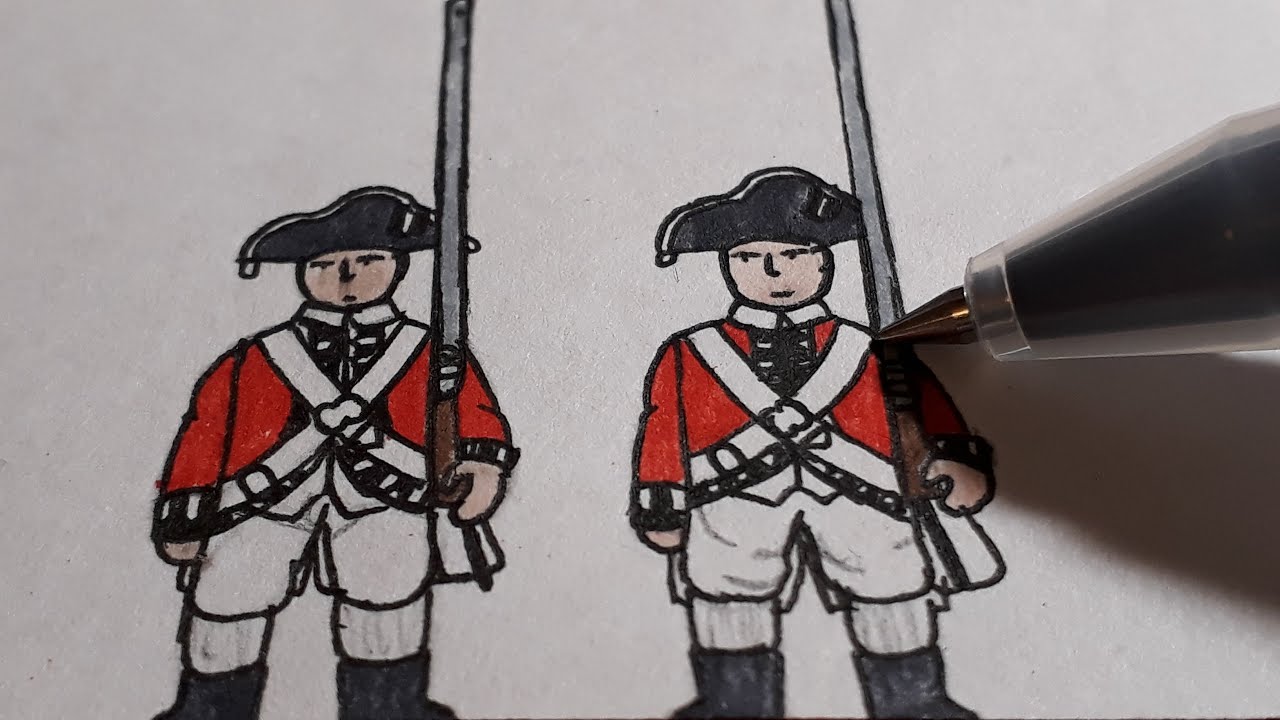The image shows a childlike, amateurish drawing of two British Revolutionary War soldiers, rendered in thick black pen and colored pens or markers. Both soldiers are depicted in red coats with black and white lapels, black tricorn hats, white knee-length pants with grayish socks, and black boots. They each hold a long musket, colored brown and silver, in their right hand. The drawing includes white suspenders and an ammunition bag slung across each of their bodies. The background of the drawing is plain white, but there is an unusual detail: the drawing is placed over what seems to be a real photograph of a machine or perhaps part of a keyboard on the left side. Additionally, a pen appears from the top right corner, as if someone is finishing the illustration.